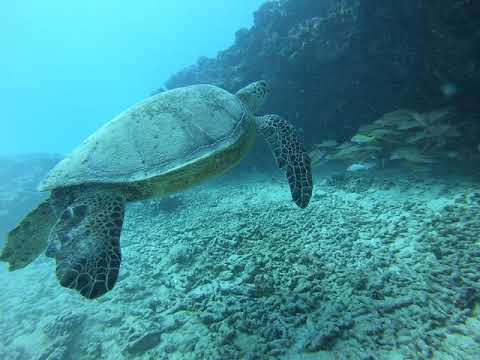The image is a rectangular underwater photograph featuring a large sea turtle as the focal point. The turtle is captured swimming to the right, viewed from its right side and slightly from the rear, showcasing its detailed green and black shell. It occupies a significant portion of the image. The background reveals a slightly foggy, light aqua-colored water, which gets clearer toward the upper left corner, hinting at the ocean's surface. The ocean floor is a textured mix of coral reefs, rocks, and plant life. Noteworthy is a vibrant school of fish swimming beneath a larger coral and rock formation in the upper right corner. The scene vividly portrays the tranquil and diverse ecosystem of the underwater world.